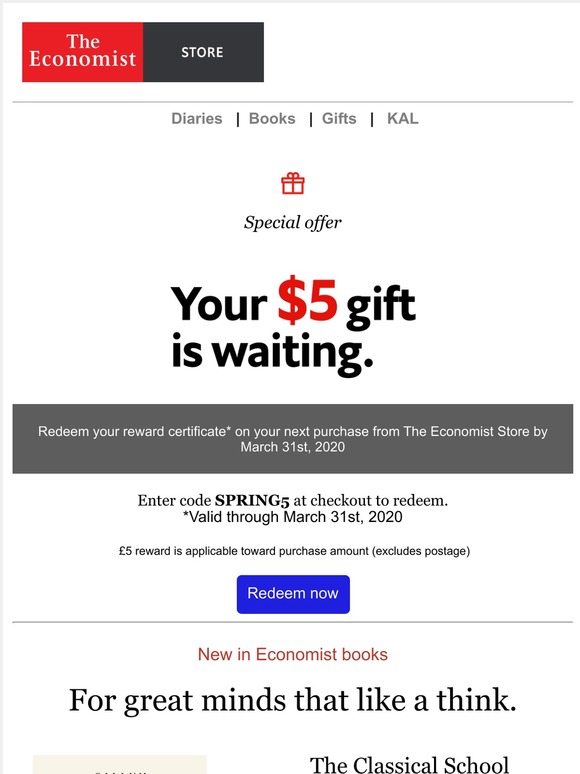Here is a revised and detailed caption for the described image:

---

The image is a promotional advertisement from The Economist store, prominently featuring the brand's signature logo at the top left: "The Economist" in white text against a bold red background. Adjacent to the logo, on a grayish background, is the word "Store." Just below this header are four category labels in a linear arrangement from left to right: "Diaries," "Books," "Gifts," and "Cal." Beneath these categories, a red present icon is displayed, accompanied by the text "Special Offer."

Centrally located in the advertisement is a compelling message: "Your $5 Gift is Waiting," with the dollar sign and the number "5" highlighted in red. Below this announcement, there's an instruction box that reads, "Redeem your reward certificate on your next purchase at The Economist store by March 31, 2020." Further details follow, indicating the redemption process: "Enter code SPRING5 at checkout to redeem. Valid through March 31, 2020."

At the bottom of this central section, another inviting box contains the call-to-action "Redeem Now," displayed in white text on a blue background. The footer of the image reads "New in Economist Books for Great Minds that Like to Think," hinting at the intellectual treasures available for purchase.